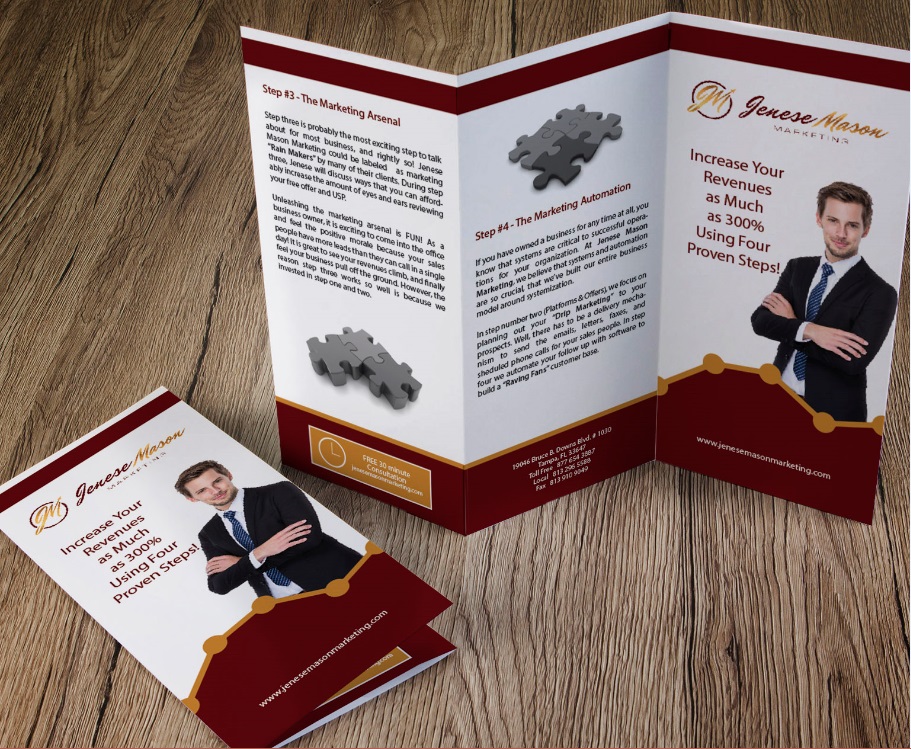The photograph captures two identical pamphlets displayed on a brown wooden table. The pamphlet on the left is folded, showing only the cover, which features a man with brown hair, dressed in a dark suit, blue tie, and white button-down shirt, with his arms folded across his chest. The cover text prominently features "Genesee Mason" in distinct red and gold font and a bold headline stating, "Increase your revenues as much as 300% using four proven steps." The pamphlet on the right is unfolded in an accordion style, standing upright to reveal its three sections: the back, the middle, and the front cover. The middle and back sections each feature an image of a puzzle and two paragraphs of text detailing step 3, "the marketing arsenal," and step 4, "the marketing automation."